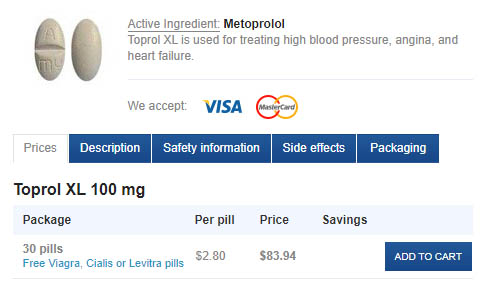The image appears to be a detailed online medication listing for a pill identified as Toprol XL, used in the treatment of high blood pressure, angina, and heart failure. The pill is depicted as an oblong, beige tablet with a score line for splitting. The front of the pill is engraved with an "A" at the top and "ML" at the bottom, while the backside is a shiny beige surface.

Prominently featured is the brand name "Toprol XL," followed by a description of its active ingredient, Metoprolol, underlined for emphasis. Annotations in gray text further describe the medication's uses. The image includes payment information, displaying the Visa and MasterCard logos. The Visa logo consists of blue text with a yellow mark on the "V," while the MasterCard logo features interconnected circles—one red and one gold—with the name MasterCard in black text.

Below the payment information, the image provides options for prices and packaging details in a structured table. Prices, description, safety information, side effects, and packaging are highlighted in white text against navy blue banners. Specifically, the table lists a "Toprol XL 100 milligrams" package, outlining prices: $2.80 per pill, totaling $83.94 for a 30-pill package. No savings information is provided.

Additional promotional offers are visible, such as free Viagra, Cialis, or Levitra pills, highlighted in blue text. A notable navy blue "Add to Cart" button invites interest in purchasing the medication, underscored with a clear call to action in white text.